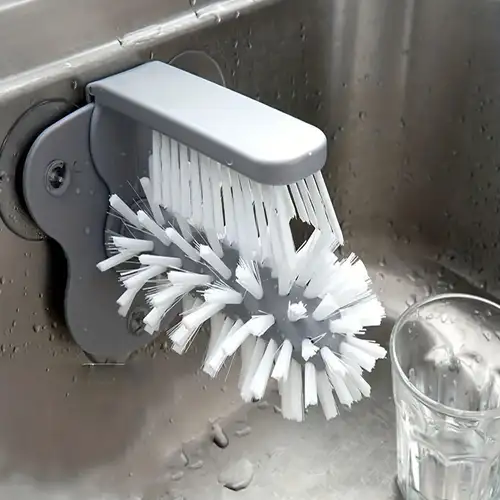The image showcases a clean, silver-gray automatic dishwasher sink equipped with an advanced cleaning attachment. The attachment features two distinct types of brushes: a white bristled, vertical brush and a cylindrical brush covered in bristles. The sink, illuminated by natural daylight, contains a transparent glass cup and scattered water droplets, suggesting recent use. The bristles on the brushes are pristine and free of food debris, emphasizing the sink's cleanliness and readiness for further dishwashing tasks.